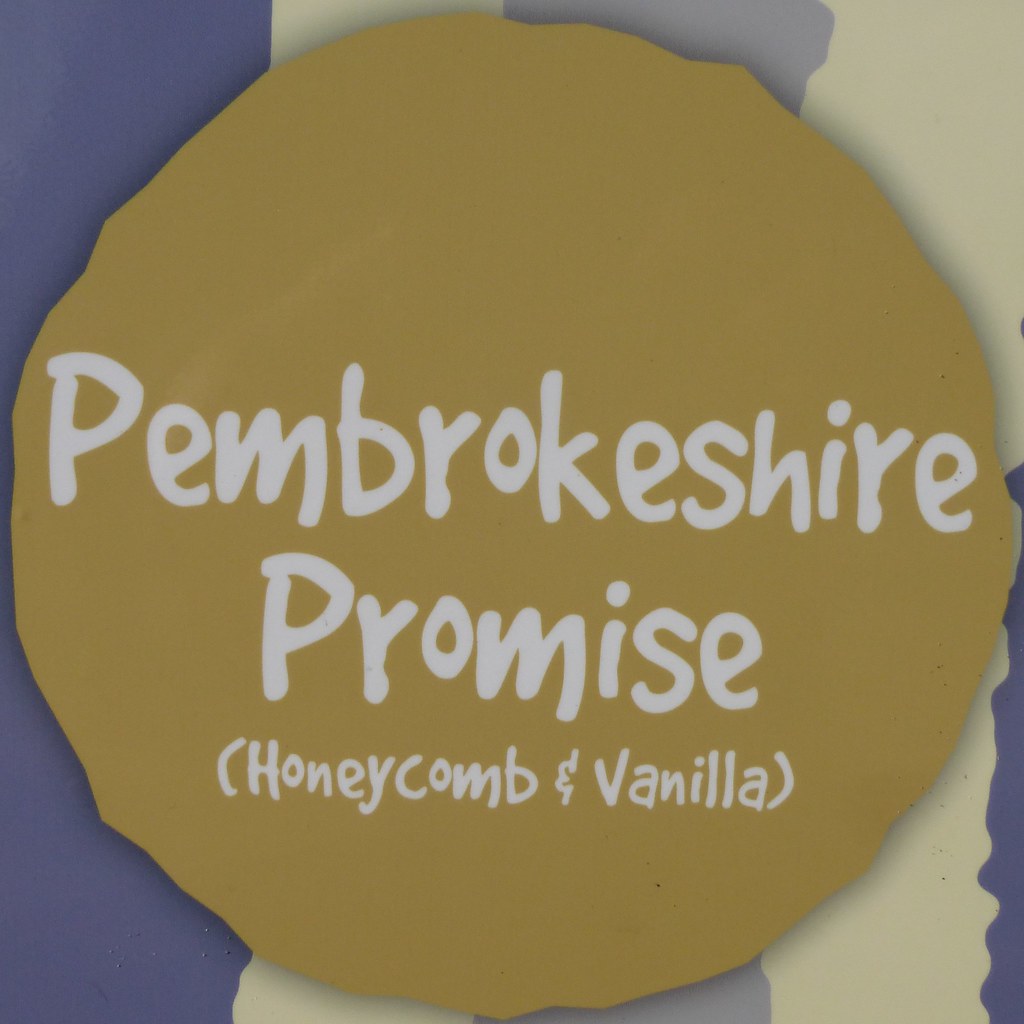A detailed close-up image features a roughly-edged, brownish circular piece of paper or sign atop a backdrop with blue and white stripes interspersed with lavender and cream bands. The brown circle, described as a brown mustard color, includes white handwritten lettering. The top word on the circle reads "Pembrokeshire," followed by "Promise," and below that in parentheses, "Honeycomb and Vanilla." The backdrop showcases a pattern with varying shades of purple, cream, and blue. The image appears to focus on this specific label, possibly indicating an ice cream flavor named Pembrokeshire Promise.